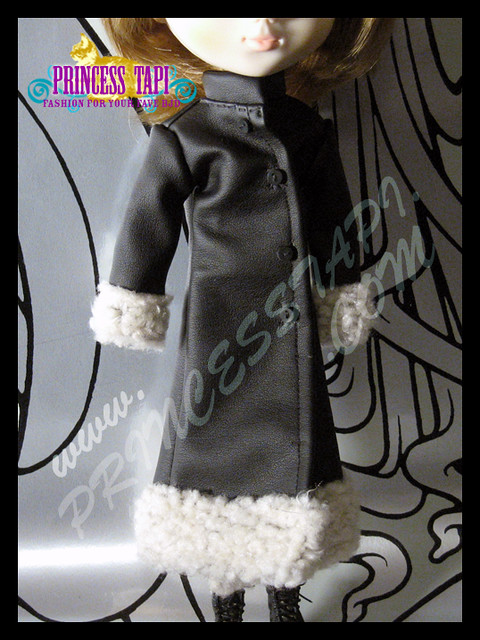A mostly vertical image features a doll dressed in fashionable attire. The doll portrays a young white girl with fiery red hair that falls just below her chin. Only portions of her face are visible, including her soft cheeks, the lower part of her nose, and her delicate pink lips. She is adorned in a chic black coat, buttoned up and accented with white fringes at the sleeves and hem. Complementing her ensemble, she wears stylish black boots. In the upper left corner, purple text in all caps reads "PRINCESS TOPPY" followed by "fashion for your," though the rest of the wording is obscured. The background has a sophisticated grayish-black design. Diagonally across the image, from the bottom left to the upper right, a script in bold lettering displays "www.princesstoppy.com."